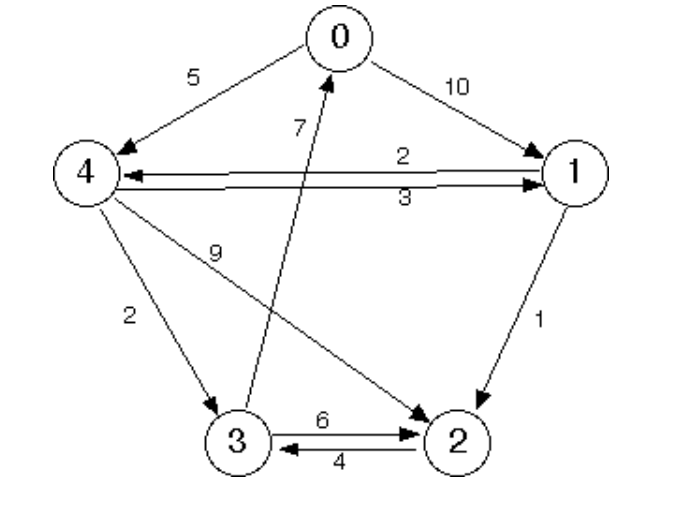This diagram appears to be an illustration used in a geometry or computer networking context, possibly representing a shortest path algorithm. The graph displays five numbered circles labeled from 0 to 4, arranged in a roughly hexagonal pattern. Each circle is connected to one or more of the other circles by arrows, indicating directed paths with associated weights. The connections and their respective weights are as follows: circle 0 connects to circle 1 (weight 10) and circle 4 (weight 5); circle 1 connects to circle 2 (weight 1) and circle 4 (weight 2); circle 2 connects to circle 3 (weight 4); circle 3 connects back to circle 0 (weight 7) and to circle 2 (weight 6); and circle 4 connects to circles 1 (weight 3) and 2 (weight 9). The entire graph is presented in black on a white background with no additional text or letters, showcasing only the labeled nodes and their connecting paths.